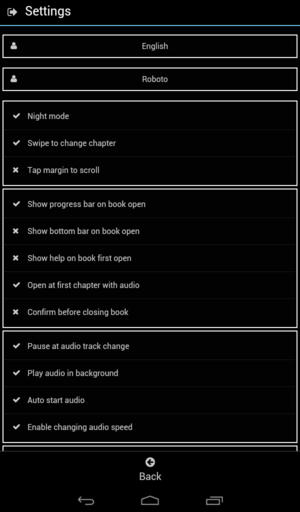The image features the settings interface of an e-reader app in night mode. The interface can be seen with the following toggles: 'Settings,' 'English,' 'Roboto,' 'Night Mode,' 'Swipe to Change Chapter,' 'Tap Margin to Scroll,' 'Show Progress Bar on Book Open,' 'Show Bottom Bar on Book Open,' 'Show Help on Book First Open,' 'Open at First Chapter with Audio,' 'Confirm Before Closing Book,' 'Pause at Audio Track,' 'Change Play Audio and Background,' 'Auto Start Audio,' and 'Enable Changing Audio Speed.' Most options have check marks next to them, indicating they are enabled, with the exceptions of 'Confirm Before Closing Book,' 'Show Help on Open,' 'Show Bottom on Book Open,' and 'Top Margin Scroll.'

At the top, near the 'English' and 'Roboto' settings, there is a white silhouette of a person, which might indicate account-related options or user profile. The bottom of the screen features navigation elements, including a 'Back' button with an arrow, another arrow pointing right, a home button, and a tab button for multitasking. This organized layout allows users to customize their reading experience extensively, ensuring optimal comfort and usability.